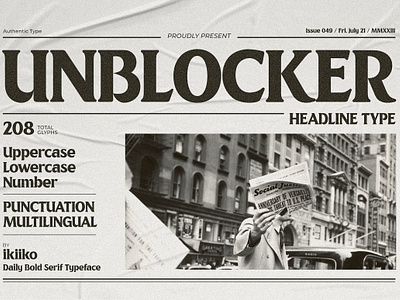This image showcases a digital mockup of a newspaper template designed to highlight a specific font. The top of the page prominently features the phrase "PROUDLY PRESENTS UNBLOCKER," followed by "HEADLINE TYPE." Below, the text details that the font includes 208 glyphs, covering uppercase, lowercase, numbers, punctuation, and multilingual options. The font, named Unblocker, is described as a bold serif typeface created by IKIIKO. The design mimics an actual newspaper format, including a placeholder for the date, shown as "Friday, July 21st" with the year in Roman numerals (likely 2022 or 2023). On the bottom right of the template, there's a black-and-white image depicting a person holding a newspaper in front of their face, set against a cityscape with tall buildings and cars, suggesting an urban environment. This mockup, complete with some digital creases mimicking real paper, serves as an advertisement to showcase the versatility and stylistic elements of the Unblocker font in a traditional newspaper setting.